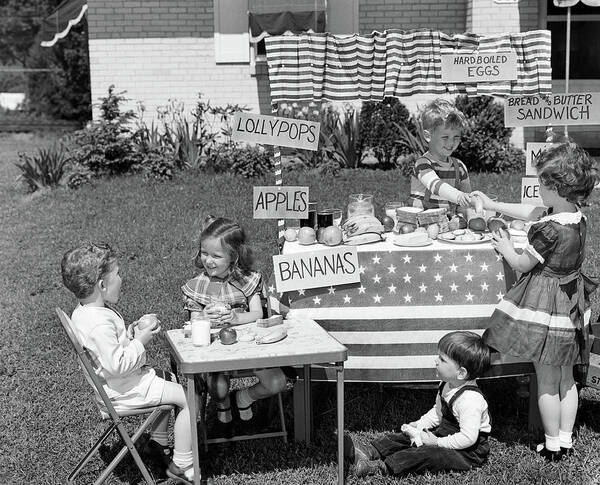This captivating black-and-white photograph, likely taken in the late 1950s or early 1960s, features a charming scene of five young children who have set up a quaint food stand on the front lawn of their home, visible in the background. The oldest child appears no older than five or six, with most around the age of three. The setup includes a toddler-sized card table draped with an American flag tablecloth, functioning as their sales counter, adorned with handmade cardboard signs advertising lollipops, apples, bananas, bread and butter sandwiches, ice pops, and hard-boiled eggs.

Two children, a boy and a girl, are seated at a small adjacent table, each holding an apple and one with a glass of milk, while a banana and another apple lie on the table next to what might be a sandwich. In front of the sales counter, a toddler, presumably the baby brother, sits on the ground. Interacting at the stand, dressed in period-appropriate attire—dresses with crinolines for the girls and a striped shirt for the boy—the slightly older boy behind the counter hands a banana to a similarly aged girl. The makeshift stand exudes a nostalgic charm, enhanced by the children's earnest expressions and the lovingly crafted signs that make this a heartwarming snapshot of mid-20th-century childhood.